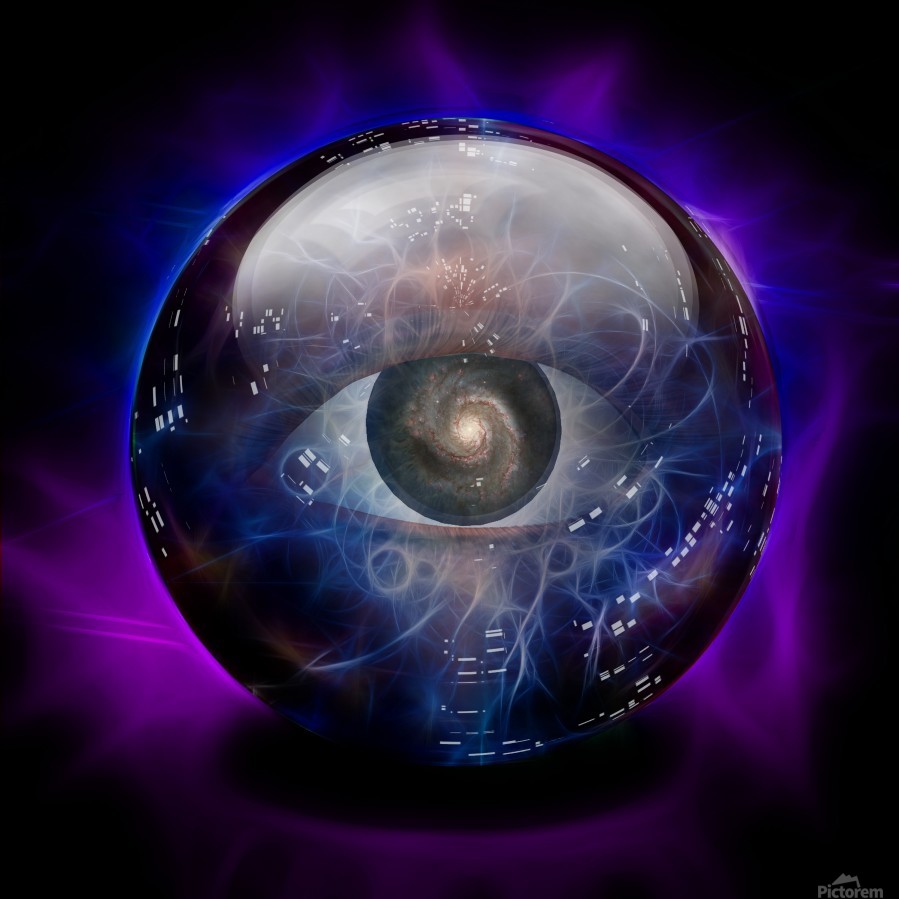The image appears to be a digitized piece of art, potentially a painting or watercolor, featuring a central, eye-like orb. The orb is predominantly purple and black, with its pupil resembling a spiral galaxy in the very center. This central eye includes a black pupil surrounded by white and various blue, brown, and white streaks and dots, adding depth and dimension. The surrounding aura extends from the orb, blending into vibrant shades of blue at the top and purple at the bottom. The entire composition is set against a backdrop that is primarily black, creating a stunning contrast that accentuates the intricate details of the eye and its energetic surroundings. The image bears the label "Pictorim," indicating the company or website associated with this artwork.